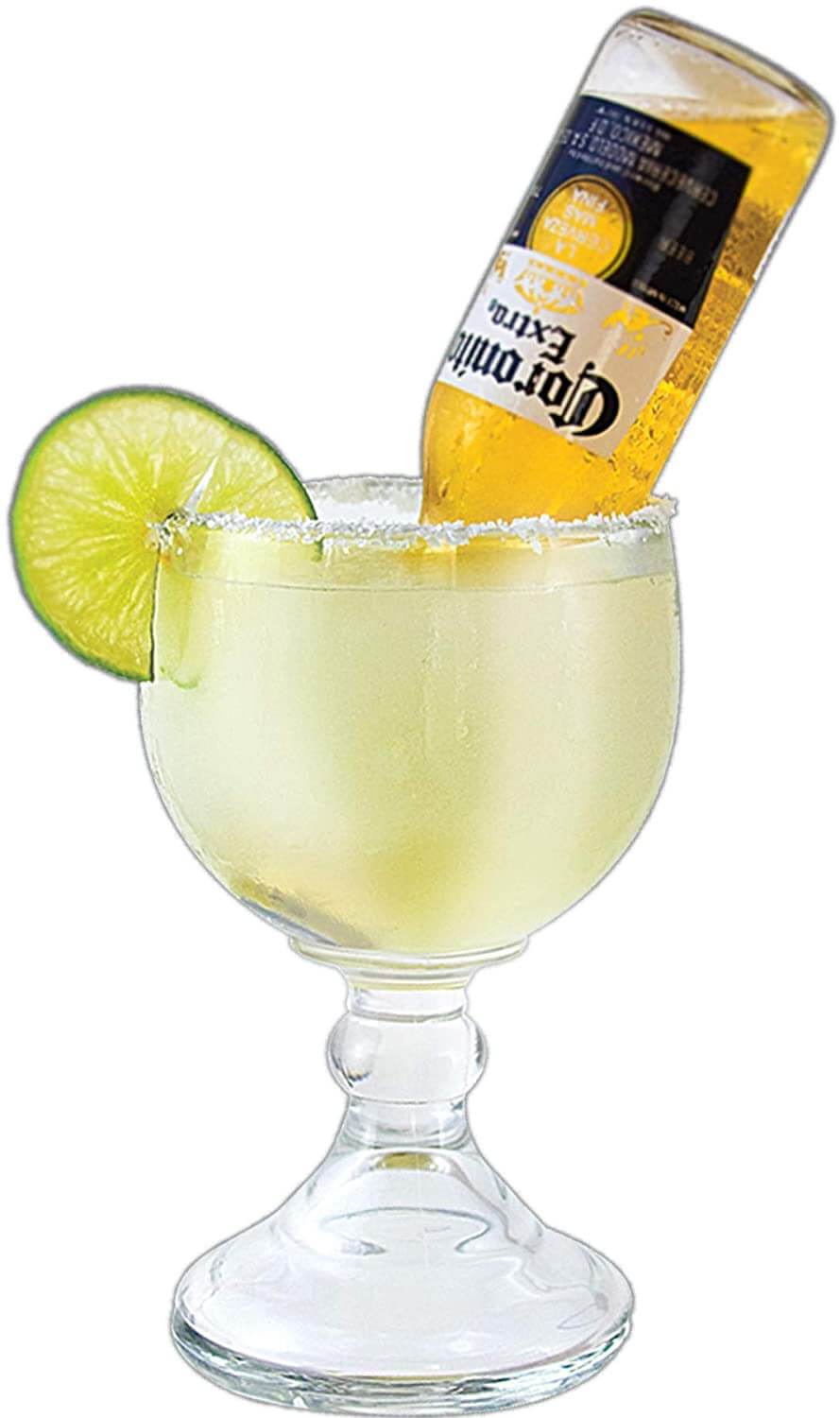The image, presumably part of a Corona beer advertisement, features a large, clear margarita glass prominently standing out against a completely white background. The glass, characterized by its broad bowl and elegant stem, has a rim encrusted with salt crystals. A perforated lime wheel adorns the glass's edge. Inside the margarita glass, there's a pale yellow liquid suggesting a classic margarita mix. Enhancing this traditional drink, a bottle of Corona Extra beer is tipped headfirst into the margarita glass. The iconic beer bottle, recognizable by its label, is partially emptied, with visible beer still inside and space at the top where the liquid is flowing into the margarita. This drink, sometimes referred to as a "trash can margarita," combines the refreshing elements of tequila and lime with the added twist of Corona Extra, a popular variant often enjoyed in Mexico.